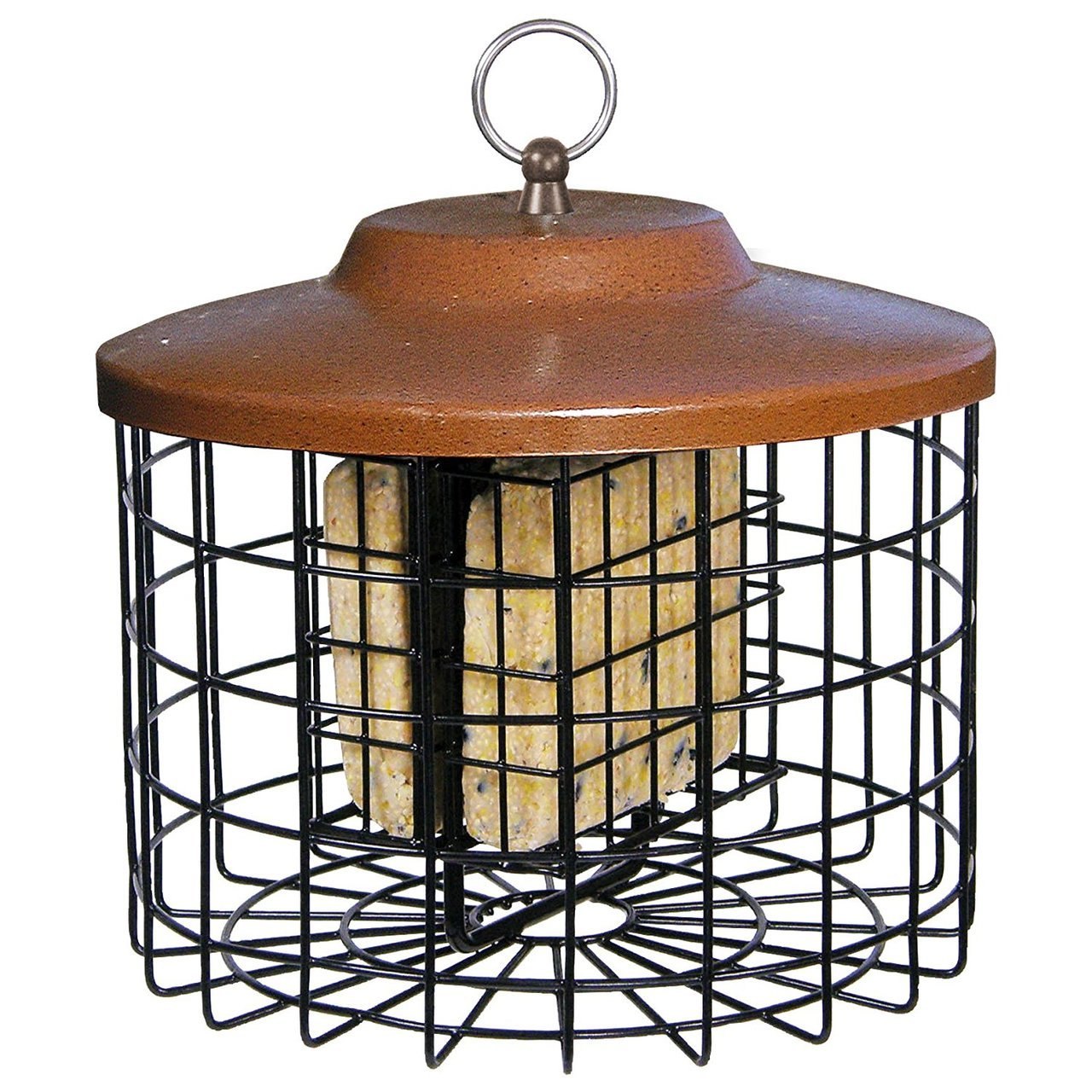The image displays a cylindrical, bird feeder-like contraption, isolated against a white background. This real, tangible object features a brown metal lid with a circular silver hook on top for hanging. The structure is a black, thin-wired cage, designed to encase and protect its core contents. Inside the cage, there is a yellowish-beige block speckled with black or blue dots, possibly mold or seeds, suggesting it is a type of bird feed or compacted seeds. The cage-like design not only holds but also guards the feed block from larger garden animals while allowing access to smaller birds.